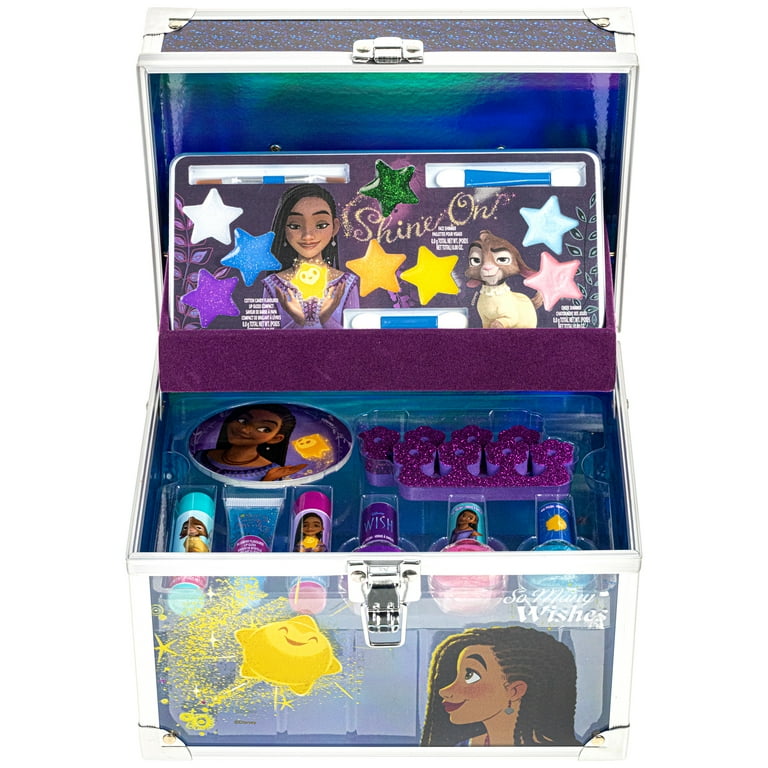The image showcases a children's makeup kit in the form of a colorful, metal storage chest with a clasp lock. The exterior features a vibrant illustration of a dark-skinned girl with dark brown braids dressed in a purple outfit, smiling, as she gazes towards a cheerful star with eyes and a smiling mouth. To the right is a whimsical character resembling a bunny goat wearing a beige outfit with a calm, smug expression. The background of the design is adorned with stars in various colors including blue, purple, pink, and yellow.

The box opens up to reveal an organized array of makeup tools and accessories. At the top, a purple drawer contains a palette with an assortment of colorful makeup including blue, green, yellow, purple, white, and pink, along with illustrations of the girl, the star, and the goat. Phrases such as "SHINE ON" are inscribed in gold lettering.

The bottom section of the box includes two toe separator sponges for pedicures, lip balms, lip glosses, and nail polishes in shades of purple, pink, and blue. The array of items also includes three brushes set among various star-shaped decorations, further hinting at the whimsical makeup theme. Overall, the kit appears delightfully tailored for children, likely inspired by or themed around a movie called "Wish."